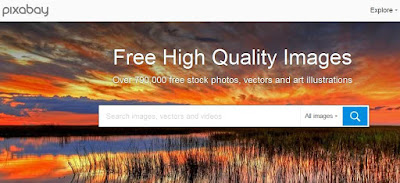The image prominently features a serene outdoor scene dominated by a captivating sunset or sunrise over a tranquil body of water. At the top of the page, a gray border houses the text "Pixabay" on the upper left corner and "Explorer" in slightly smaller text on the upper right corner. The vibrant sky is a beautiful blend of mingled colors, including shades of orange, yellow, blue, and whitish hues, with scattered clouds adding texture to the scene. The calm water below mirrors the colorful sky, enhancing the tranquil atmosphere.

In the foreground, some plants add a touch of natural detail. Overlaying the picturesque landscape, white text reads, "Free high-quality images." Below this, slightly blurry text says, "Over 790,000 free stock photos, vectors, and art illustrations." Dominating the lower portion of the page is a rectangular search bar spanning most of the width. The bar has a white background with the placeholder text "Search images, vectors, and videos." To the far right, additional text reads "All images" accompanied by a downward-pointing arrow. Adjacent to this, set against a blue background, is a white magnifying glass icon.